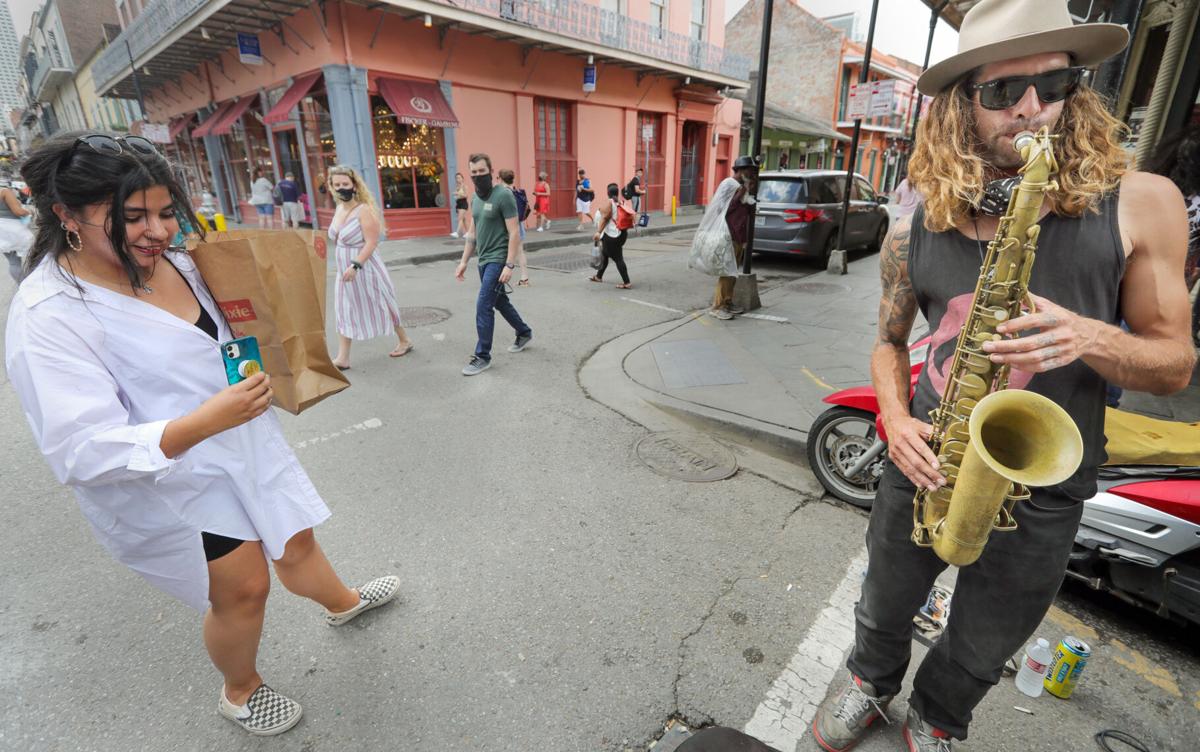The photograph captures a lively daytime street scene, framed horizontally, featuring a bustling city intersection. Dominating the right side of the image is a mid-20s to 30s white man with a fair complexion and long, curly, blondish-brown hair. He sports a beige hat, black sunglasses, a black tank top, black pants, and gray and red shoes. He is passionately playing a yellow saxophone, drawing the attention of passersby. His right arm is adorned with a tattoo, and his fingers on the left hand feature colored fingernails. Nearby on the ground, there are items like beer and water bottles, along with a parked moped.

To the left stands a captivated woman snapping a photo of the musician with a blue iPhone. She has black hair and wears a long, white button-up shirt over a black undershirt, paired with black shorts and black-and-white checkered shoes. She holds a pixie brown bag in one hand, indicating she might have just come from shopping. Sunglasses rest on her head, adding to her casual yet stylish look.

In the background, a mix of masked and unmasked individuals move through the scene, reflecting ongoing COVID-19 precautions. A couple, both clad in black masks, can be seen walking past what appears to be a cafe or restaurant, identified by the indistinct text on its facade. Overcast skies cast a soft, diffused light over the gray streets and sidewalks, encapsulating a typical yet vibrant urban moment.